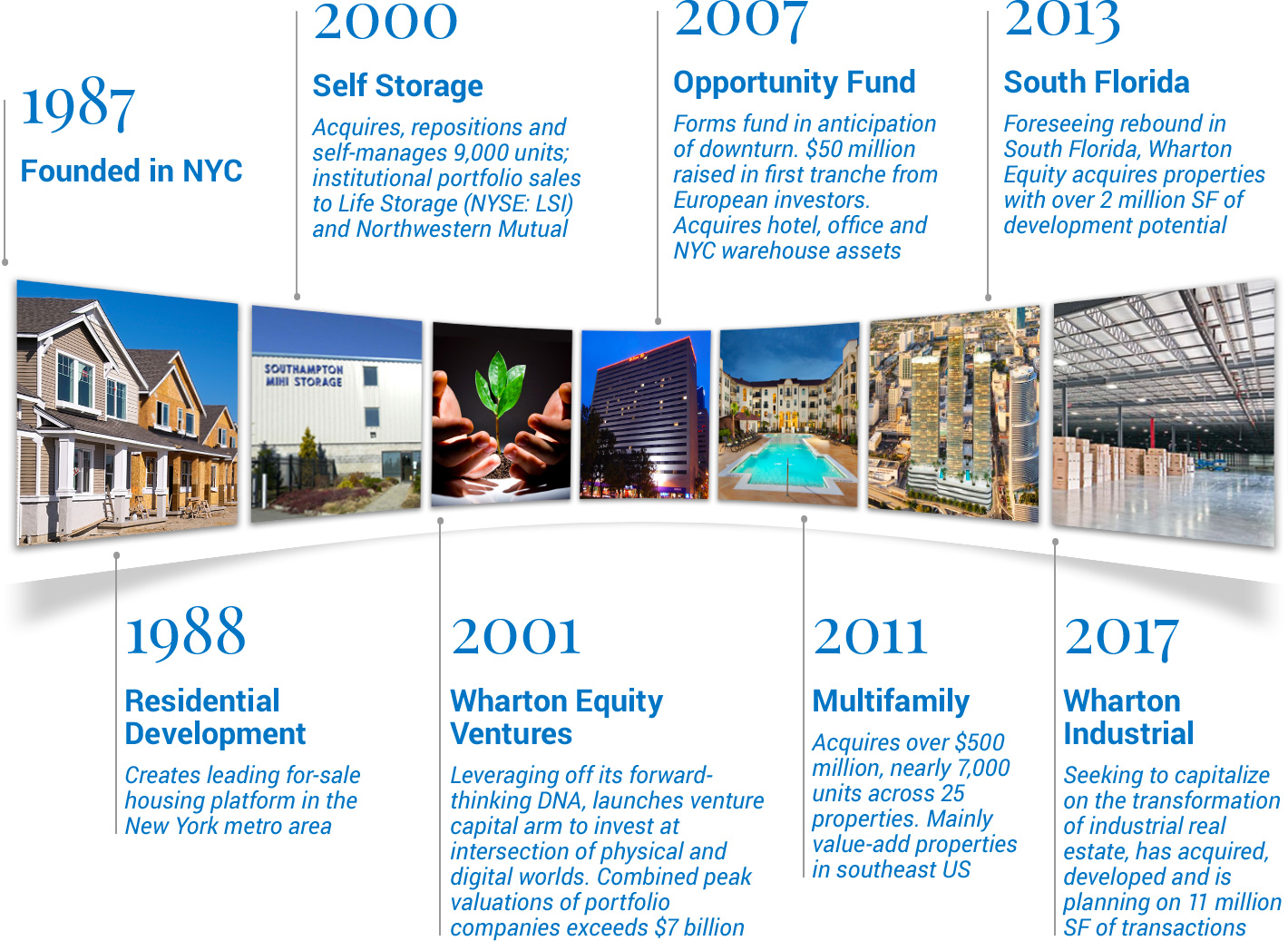The image depicts a meticulously crafted timeline starting from the left side with the founding in New York City (NYC). The timeline progresses through significant years, specifically marking 1987, 1988, 2000, 2001, 2007, 2011, 2013, and culminates in 2017, which mentions Wharton Memorial or Wharton Industrial. In the center of the image, there is a collage of various pictures, each corresponding to the key years noted on the timeline. Each photo visually represents significant events or milestones from the respective years, creating a vivid historical narrative.